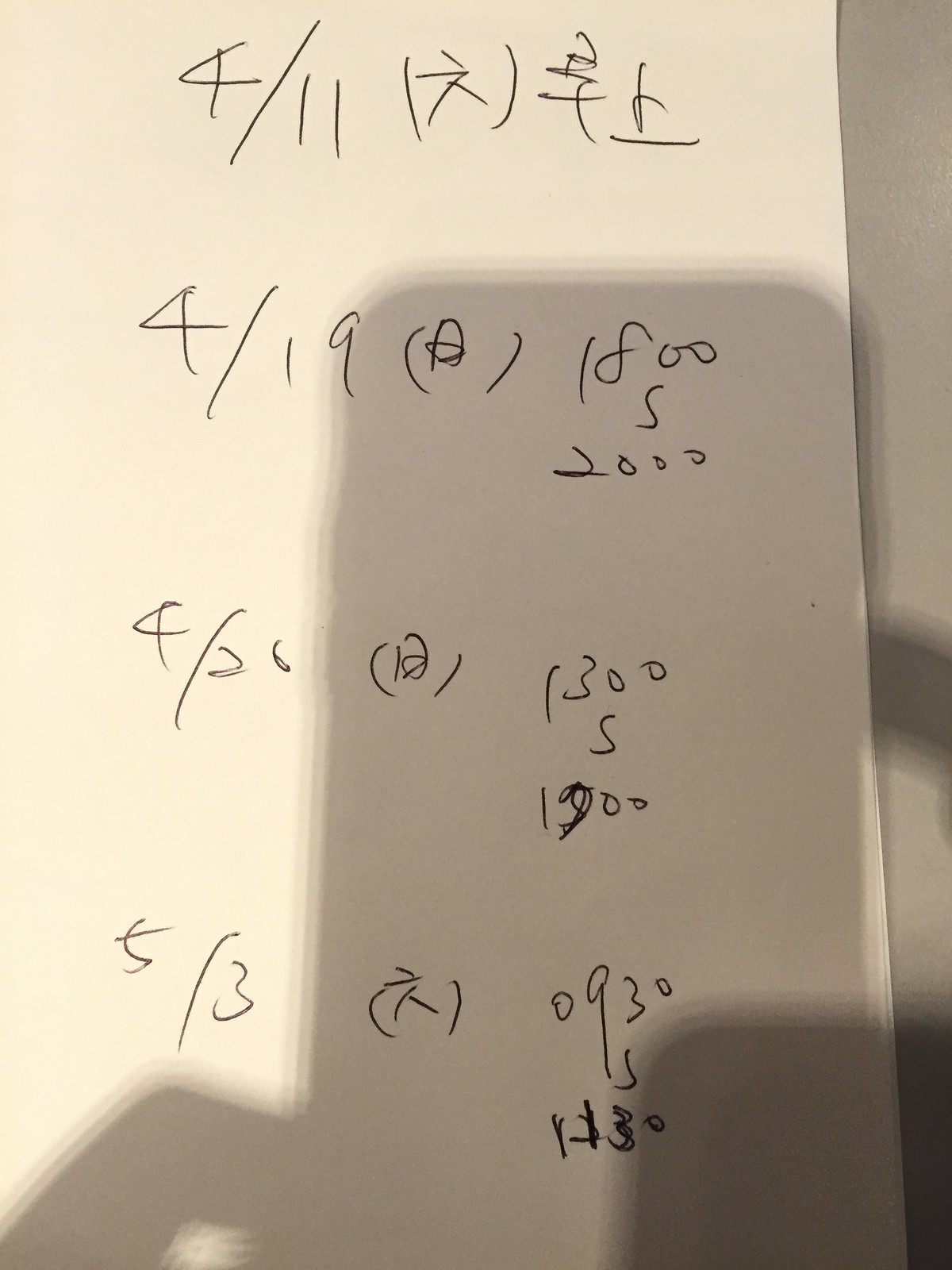The image showcases a piece of paper photographed at an angle, with a distinct shadow cast by a cell phone and fingers suggesting the image was taken with a handheld device. The photograph is tinted green. The paper contains text in what looks like Chinese, interspersed with various dates and numbers. The dates include "4/11" and "4/19" followed by Chinese characters, and a sequence of numbers "180052000 4/26," along with "1300 5," "1200," and "5/3," with further numerical details "0930 5130" written. All numerical and textual elements are in black ink. On the right side of the image, part of a dark grey surface is visible, adding contrast to the composition. The paper is skewed, not perfectly aligned within the frame, giving a casual and impromptu feel to the photograph.